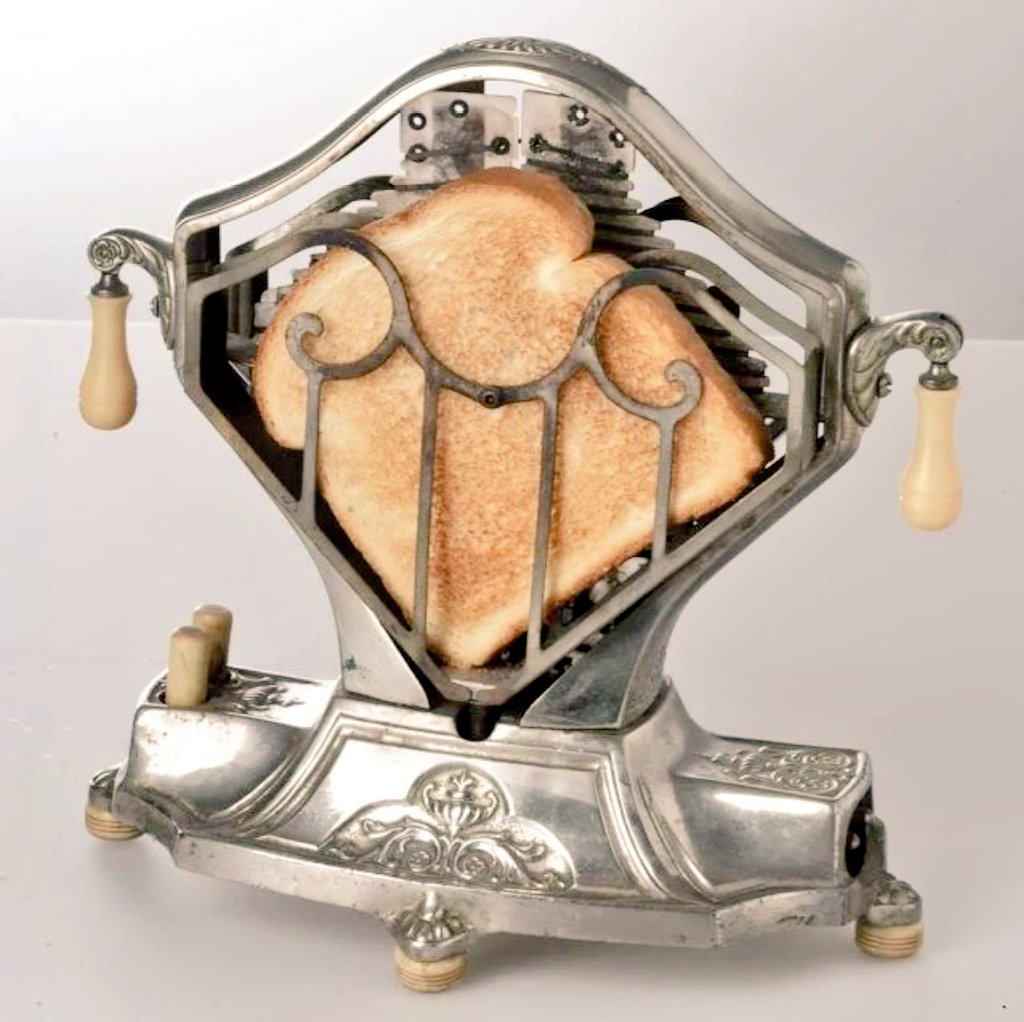The large square image depicts an antique toaster prominently positioned on a light gray countertop, with a slightly darker gray wall in the background. Natural light streams in from the upper left corner, casting a gentle glow on the scene. The toaster, crafted from metal with intricate decorative designs, rests on at least three wooden pegs that elevate it from the surface. Its front face starts as a diamond shape but curves at the top, lacking the top point of a complete diamond. Adjacent to this face are two light beige, wooden knobs on either side, designed for cranking. The toaster features a vertical slot where a piece of lightly browned toast is visible, held by old-fashioned metal bars. Behind the toast, heating elements can be discerned, showcasing how the bread is toasted. The overall appearance of the toaster, with its elaborate metalwork and antique design, suggests it might be on display in a setting like an auction house or for sale as a collectible antique.